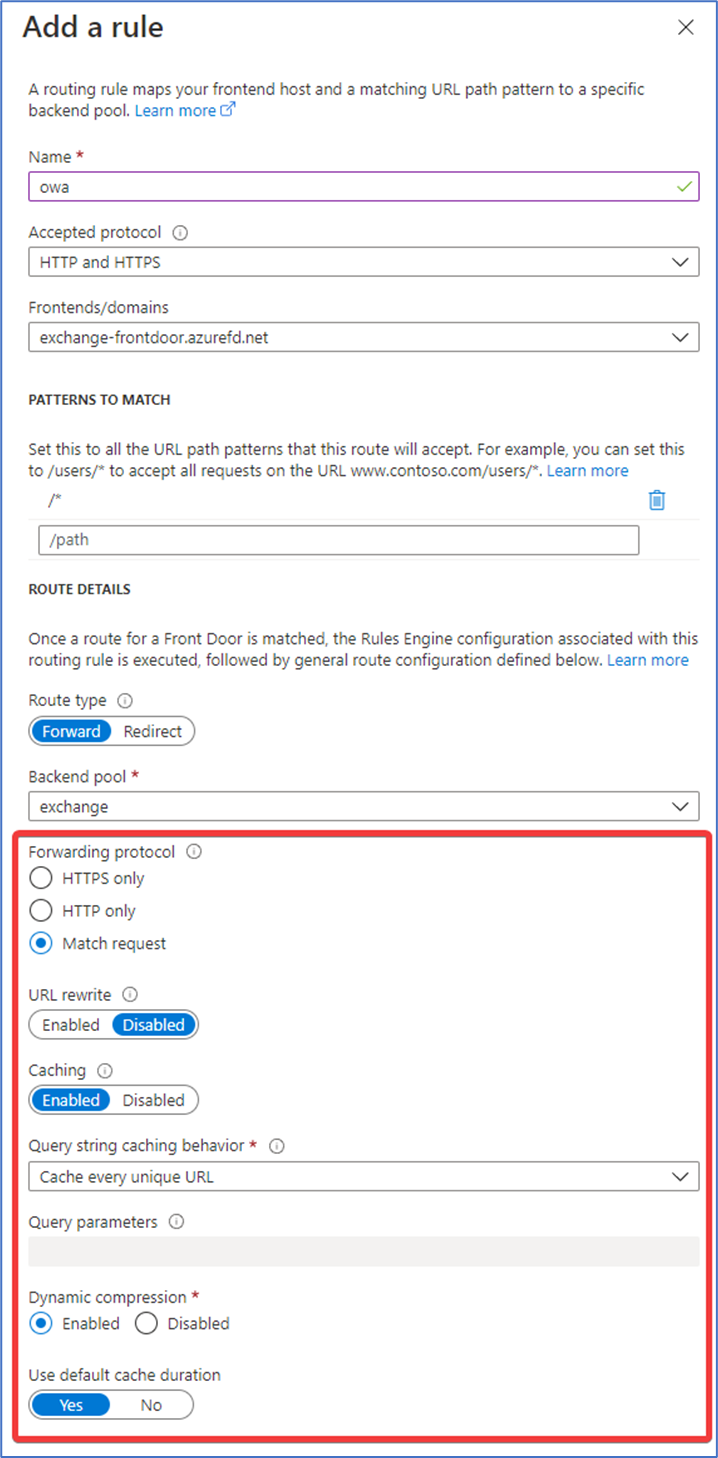This rectangular image, oriented with its longer side extending vertically, is bordered by a thin blue line. At the very top, in a prominent font size, the image displays the word "Adderall". Positioned in the upper right corner, there is an "X" symbol. Directly below the title "Adderall," the text reads: "A routing rule maps your front-end host and a matching URL path pattern to a specific back-end pool."

Beneath this, the phrase "Learn More" is highlighted in blue font. The subsequent line reads "Name" accompanied by an asterisk, indicating a required field. Within the corresponding box, the word "OWA" is displayed, complete with a checkmark situated on the right side. Next in the list is a section titled "Accepted Protocol," which contains a box below it displaying "HTTP and HTTPS" along with a drop-down menu located at the far right.

Continuing downward, the title "Frontends / Domains" appears, followed by "Exchange-Frontdoor.azurefd.net," which also has a drop-down menu on the far right. Further down, the image features another section labeled "Patterns to Match," which provides the guidance: "Set this to all the URL path patterns that this route will accept. For example, you can set this to /users/* to accept all requests on the URL www.toso.com/users." The phrase "Learn more" appears again, inviting further exploration of the information provided.